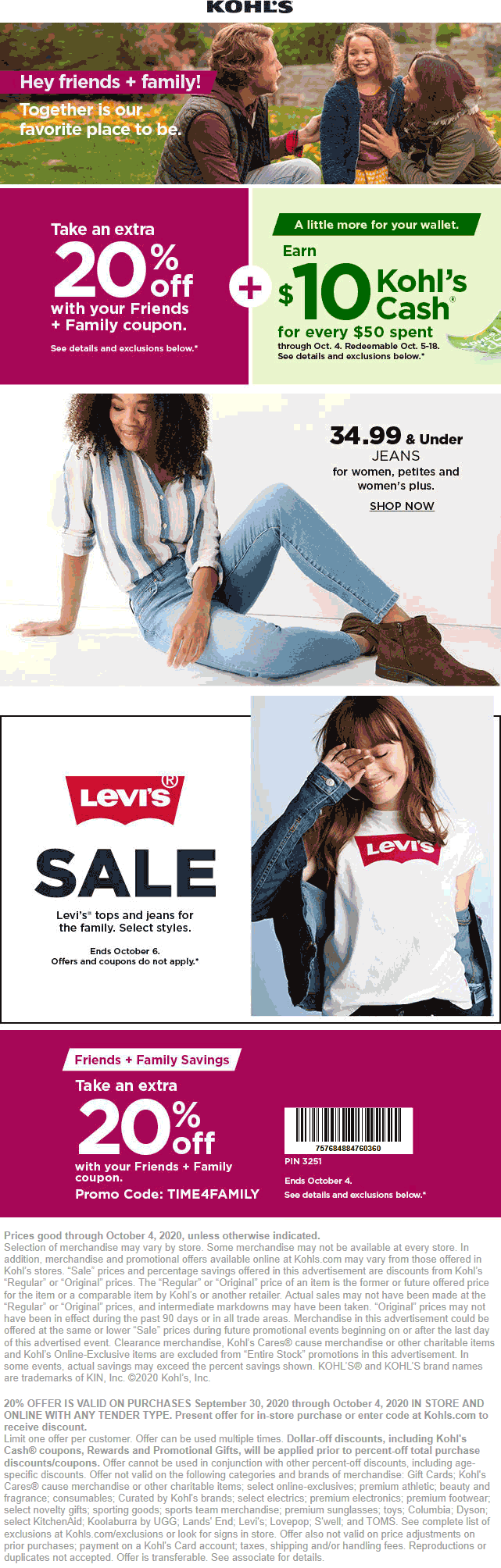This image is a detailed screenshot of a Kohl's advertisement. At the very top, a white rectangle features the Kohl’s logo in bold black font. Directly below, a graphic depiction showcases a Caucasian family of three—a man, a little girl, and a woman—kneeling together in a grassy area. To the left of the man's head, text in white font reads, "Hey friends and family, together is our favorite place to be." Beneath this, a mauve square displays a message in white font: “Take an extra 20% off with your friends and family coupon.” Adjacent to it, a beige square includes text stating, "Earn 10 Kohl’s Cash for every $50 spent."

Below this section, another advertisement features an African American woman in her early 20s, lying on the floor. She has long, fluffy hair and is smiling towards the left. She is dressed in a white and blue top paired with tight, light blue jeans and brown boots.